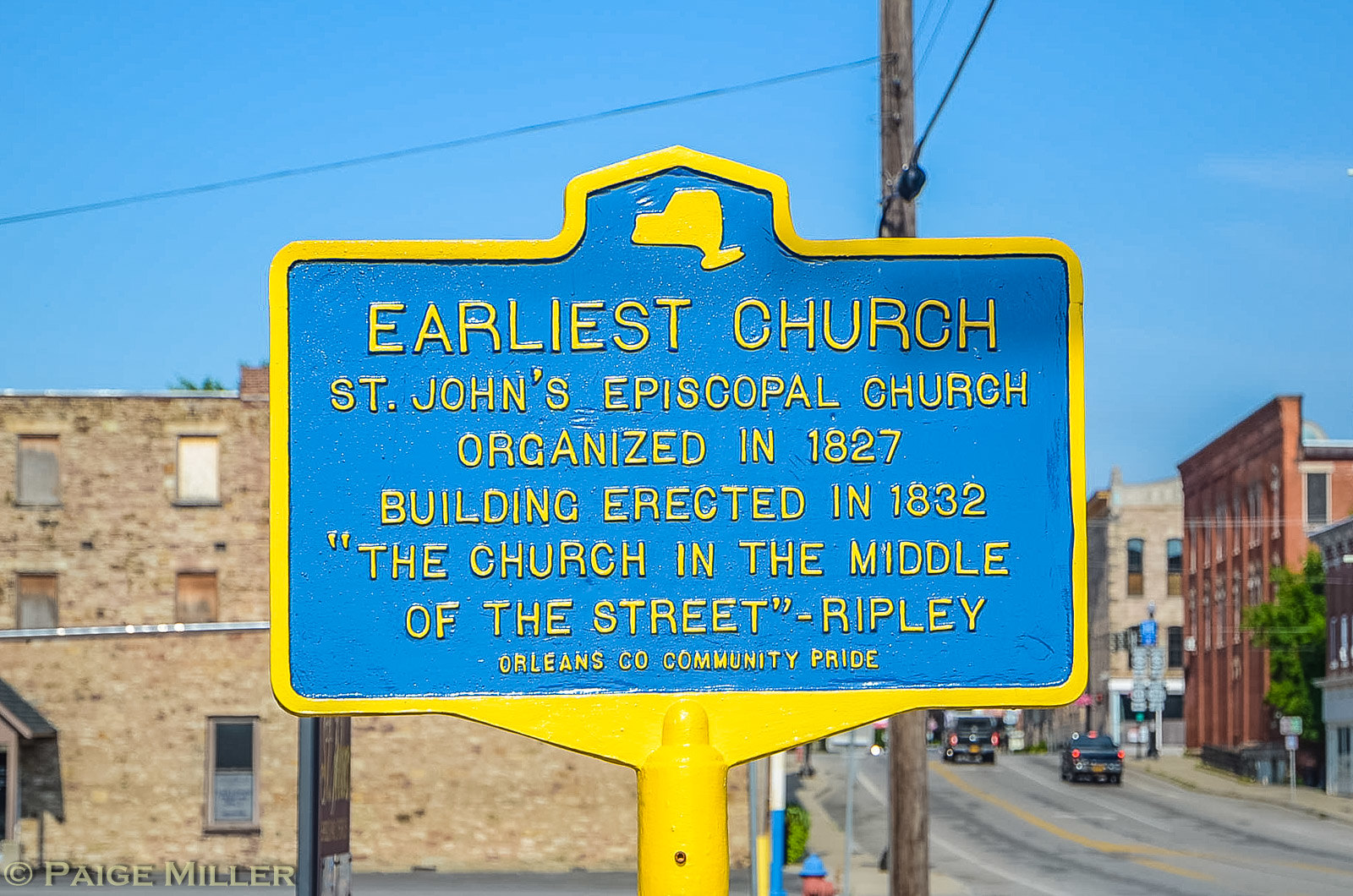In front of a serene blue background sits a historic, small-town cityscape, featuring three-story brick buildings that exude charm without towering height. A prominent metal sign stands in the foreground, distinguished by its light blue face and contrasting yellow border, which extends to the round metal post supporting it. Embellished with a yellow outline of New York State at the top, the sign reads in bold yellow letters, "Earliest Church - St. John's Episcopal Church. Organized in 1827. Building erected in 1832. 'The church in the middle of the street' - Ripley. Orleans County Community Pride." This testament to local history is situated near an array of power lines, and a weathered, gray stone building, adding to the rustic ambiance of the street, indicative of a historic town center.